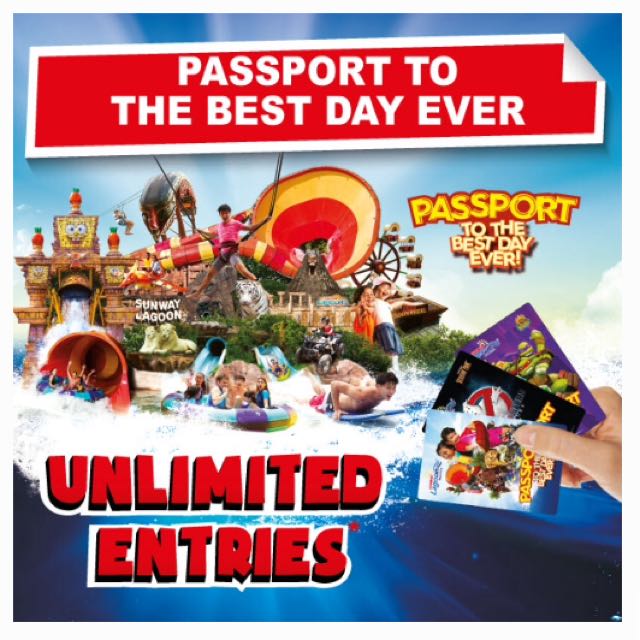The image features a vibrant blue rectangle as the background. Dominating the top of the rectangle is a bold red banner, elegantly trimmed with white edges. Within this banner, white letters spell out the phrase "Passport to the Best Day Ever." Toward the bottom of the rectangle, text in striking red letters with a white outline announces "Unlimited Entries."

On the right side of the image, a hand is holding a set of cards, each labeled "Passport." The visible cards showcase popular themes, including Ghostbusters, Teenage Mutant Ninja Turtles, and what seems to be a manga show.

The central portion of the image, situated beneath the red banner and above the bottom text, visually narrates an exciting scene from an amusement park. The park appears to be Sunway Lagoon. Depicted are people joyfully descending a water slide, presided over by a statue of a Spongebob character at the top. To the right, a person in a harness is captured mid-air, seemingly gliding, though the parachute or supporting mechanism is out of view. The scene is bustling with activity, featuring a lively beach where people are surfing and smiling, all within a setting of sparkling blue water.